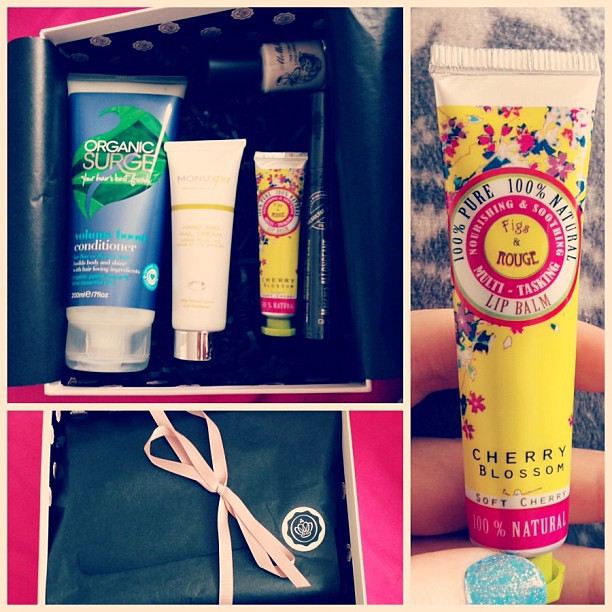The image features three distinct sections illustrating various beauty products. On the right-hand side, a tall, rectangular image showcases a cherry blossom lip balm labeled "Soft Cherry." The product claims to be 100% pure and natural. The lip balm tube is yellow, adorned with red and blue floral patterns, and is held delicately between a user's fingertips.

In the lower left-hand section, a gray box or bag is tied with a narrow pink ribbon. A small logo featuring a crown is visible on the right-hand side of the bag.

Directly above this gray box is an open container displaying four different beauty products. The leftmost item is labeled "Organic Surge," appearing to be a conditioner. Placed in the middle is a white tube. To the right of this white tube, another yellow lip balm, identical to the one in the initial image, is visible. Above it, there is a bottle of beige nail polish. The arrangement offers a detailed and visually appealing display of the beauty items.